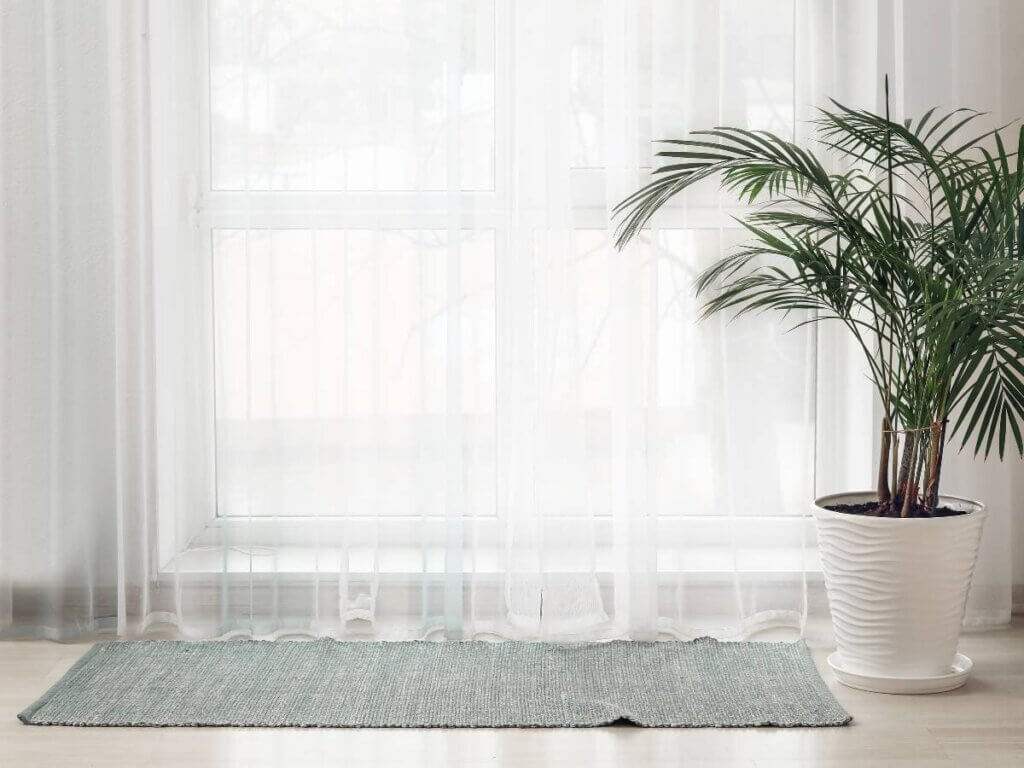The image captures a serene interior scene dominated by a bay window in a home or apartment. The window is adorned with sheer, white gossamer curtains that allow light to gently filter through, casting a soft glow across the room. Situated in front of the window is a light brown table, upon which rests a white ceramic pot featuring a subtle, wavy texture. The pot houses a tall, leafy green plant, identifiable by its long, thin leaves and brown stem nestled in dark soil. Underneath the table is a gray or light green rug, reminiscent of a small area rug or yoga mat, which rests upon a beige hardwood floor. The overall composition highlights the tranquil, airy atmosphere of the space, with the soft interplay of natural and decorative elements creating a harmonious setting.